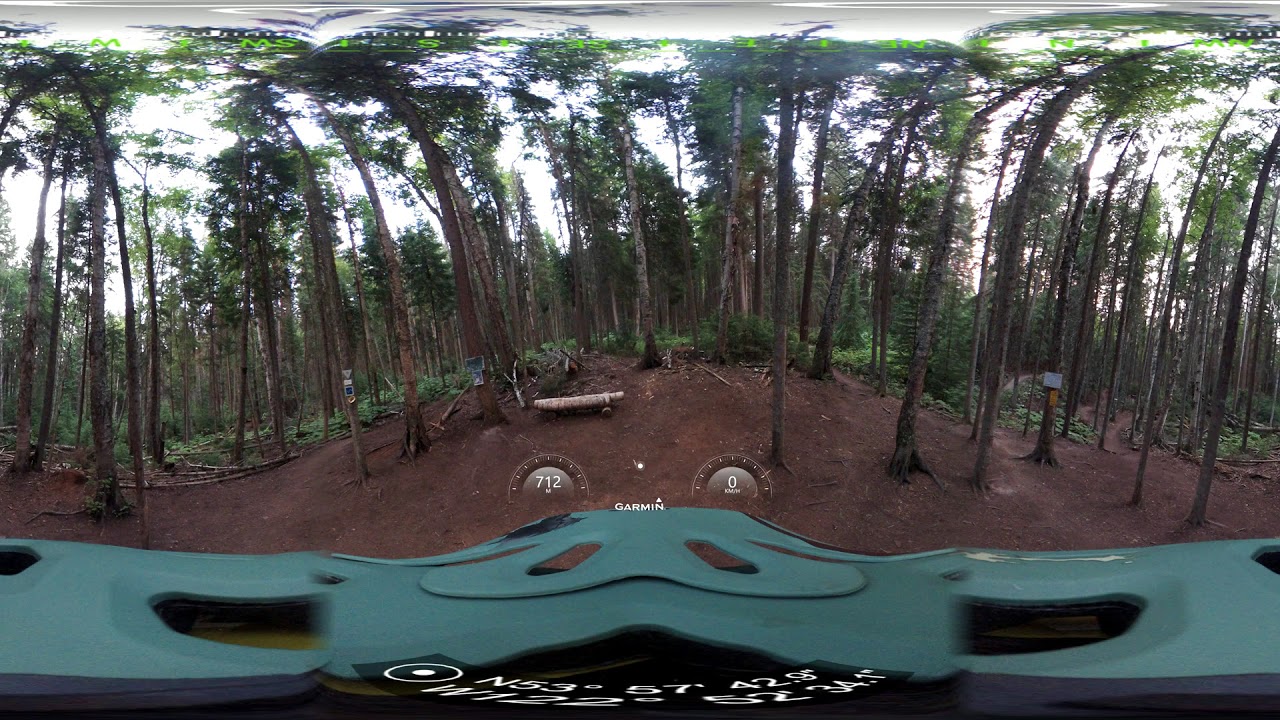The photo, taken from a camera attached to a turquoise motorized vehicle, shows the vehicle's blue-green dash occupying the bottom portion of the image. Longitude and latitude coordinates are displayed over the dash but are too blurry to discern. Centrally located at the bottom are two pedometers with the numbers 712 on the left and 0 on the right, flanking the word "Garmin" in white all-caps text. The image has a distinctive distortion at both the top and bottom, suggesting it was captured with an ultrawide or 360-degree lens. In the background, a dense forest of thin trees, resembling cedars, creates a canopy that almost obscures the sky. The trees are blurred and bent to the side, possibly due to an effect placed on the image, adding to the surreal atmosphere. There is also a hint of light yellow sunlight filtering through the canopy. The ground is mostly dirt, and the entire scene exudes a calm, relaxed vibe.